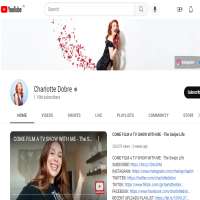The image features the homepage of a YouTube channel with two distinct sections. The upper section displays the YouTube interface with notably poor resolution. In the top-left corner, the YouTube logo appears in red. To its right is a search bar, and on the far-right is a square icon with a plus symbol, although the details are unclear.

Below this, a large photograph showcases a woman, who appears to be singing. She is dressed in a black dress and has long red hair. Behind her, there seems to be red and gray confetti, set against a white background with a noticeable white drop shadow. The name "Charlotte Dobre" is visible next to her image, suggesting that this is the homepage of her YouTube channel. Her profile photo icon is also visible next to her name.

At the top of the page, there is a navigation bar, but the text is unreadable due to the poor resolution. Further down, a video thumbnail features the same woman with red hair, wearing a black shirt. White text overlays the video thumbnail, but the content is illegible. The right side of the screen contains more information about the video, but again, the poor resolution renders the text unreadable. The overall background of the page is predominantly white.